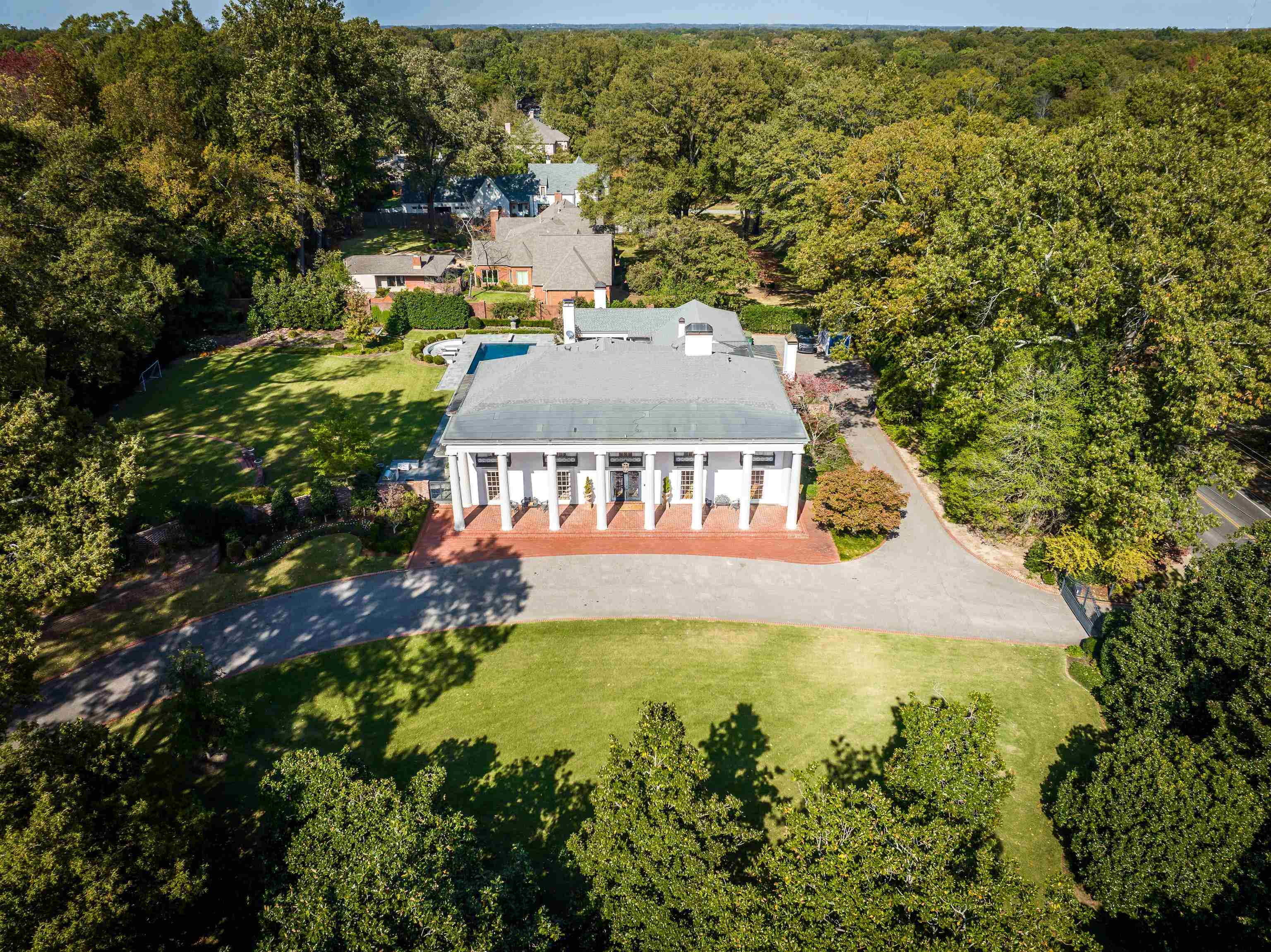This image presents an aerial view of a large white house marked by its stately facade featuring eight impressive white columns. The house has a light gray roof with two chimneys protruding from it. The arcade area of the house is constructed with red brick, adding a rich contrast to the otherwise white walls. In front of the house lies a meticulously groomed lawn and a gray horseshoe-shaped driveway that also extends around to the back. The porch stands out with its distinctive orange color.

Behind the main house, there's an in-ground, square-shaped indoor swimming pool with blue water, encircled by a gray sidewalk. This aquatic feature sits against a backdrop of dense green trees that stretch across the upper right and top of the image, illustrating the property's remote and heavily wooded location. A gated entrance leads to the driveway which features a slight dip where it extends off the image to the right and left. 

The area surrounding the house is lush with greenery, including a large green field to the right and multiple other houses in the background. One of the neighboring houses is brick-faced with a gray roof, maintaining the elegant aesthetic of the area. The scene is bathed in sunlight, casting the shadows of the trees on the ground, while a dark blue-gray sky looms in the back, adding depth to this picturesque setting.